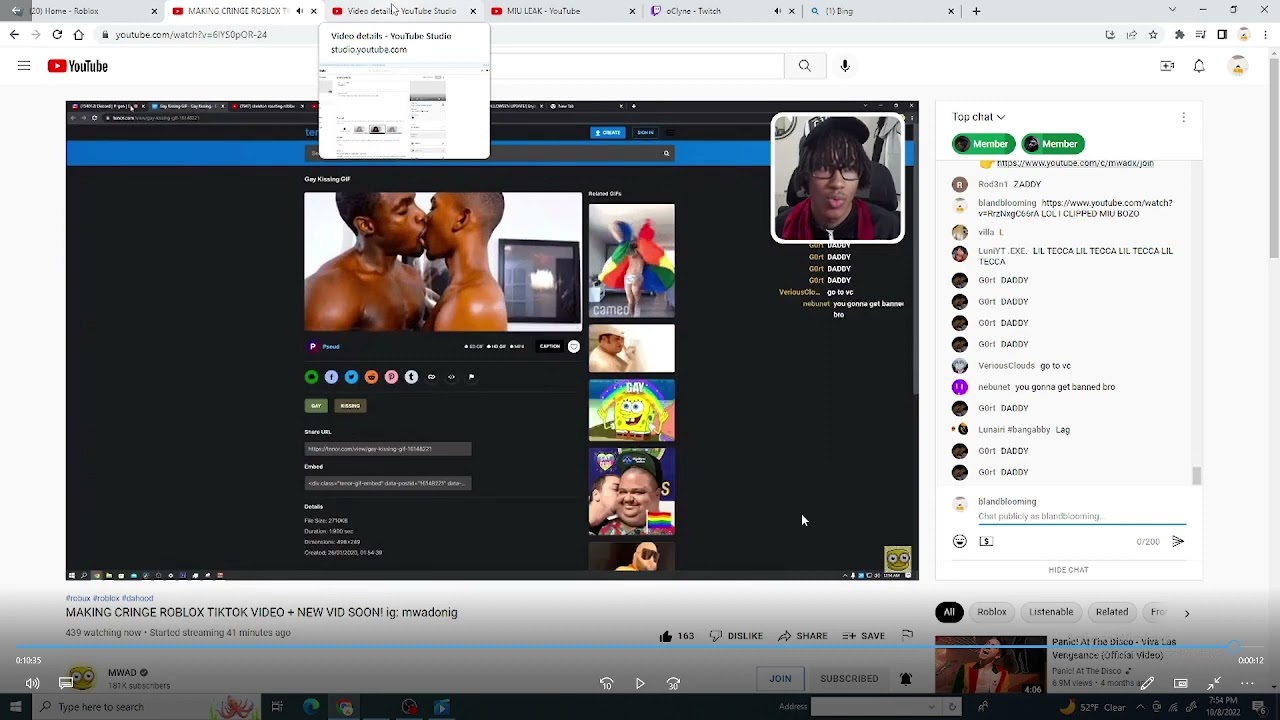The screenshot captures a full desktop view with an open YouTube page as its focal point. The highlighted video, set against a black background, features two Black men kissing, indicating the nature of the content as somewhat intimate or potentially provocative. In the upper right corner of the screen, a small overlay reveals a live stream or conference call, possibly a Zoom meeting, where two individuals are engaged in a discussion about the video. The desktop shows five other open tabs, one notably for online shopping, indicating the user is multitasking. To the far right of the image, the YouTube live chat is actively streaming comments and reactions from other viewers who are also watching the same video.